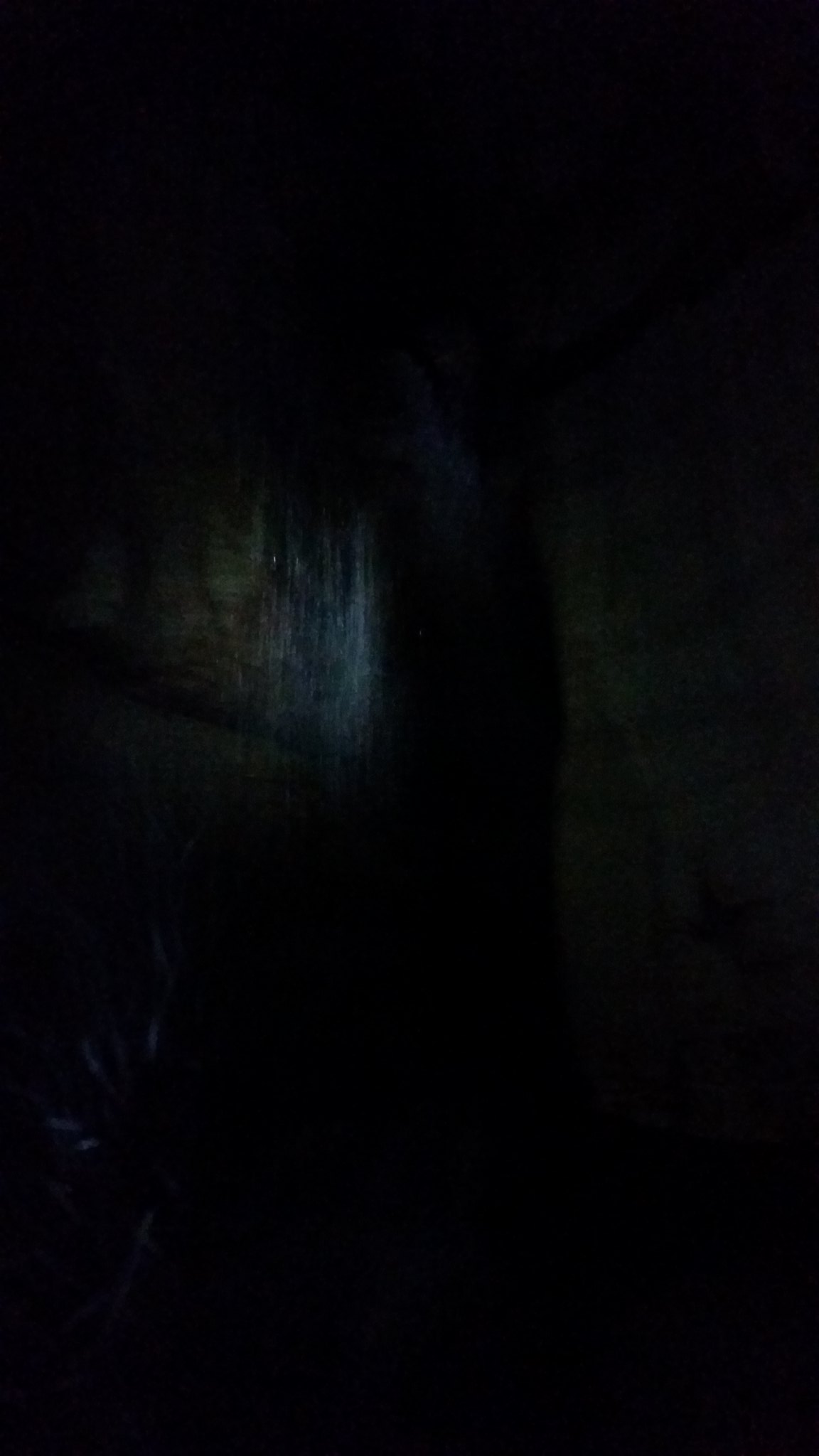The image is predominantly black and appears rectangular in shape. Near the upper middle-left side, there's a distinct streak—whitish in color—that looks like it ascends from the bottom at an angle. This streak has a faint hint of green along its left edge, and it transitions from being more solid at the bottom to a feathered pattern as it goes upward, resembling a brush stroke or a smear. The rest of the background is entirely black, with no other discernible colors or elements, making it difficult to identify any specific objects or scenes within the image.